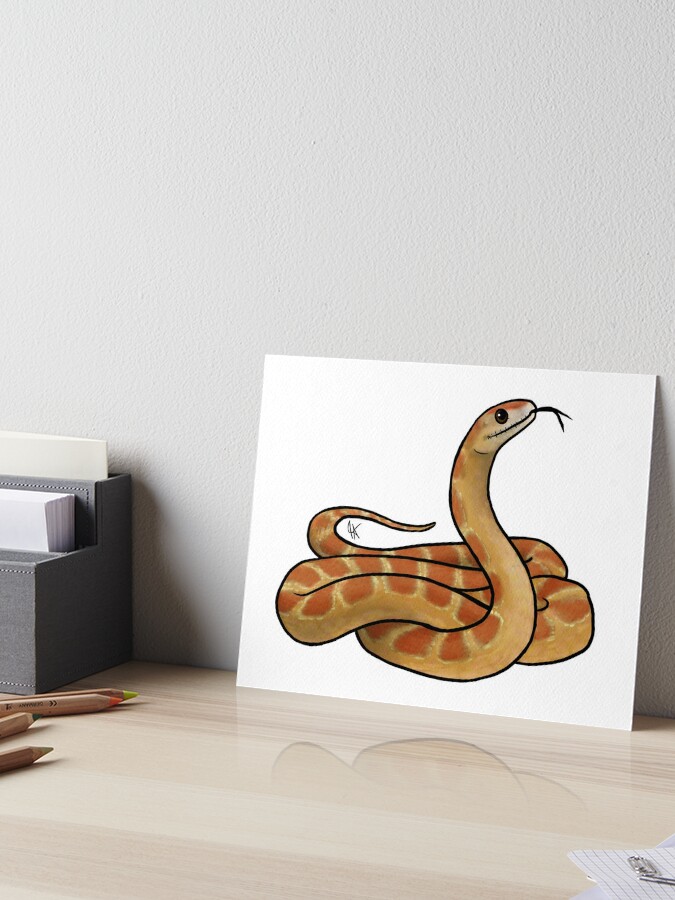In this AI-generated image of a well-lit room, a light wooden table, sanded and finished to retain its natural texture, serves as the focal point. At the center of the table is a white canvas adorned with a highly detailed drawing of a curled, light brown snake with dark brown spots. The snake's head is raised, revealing a keen brown eye and a tongue extended in a V shape. To the left of the table, a gray container holds various pieces of paper, in front of which lie four distinct colored pencils with tips in yellow, orange, green, and beige hues. These pencils are unique in that their wooden exteriors don't match their vibrant tips and bear engravings to indicate their colors. Towards the bottom right of the image, a piece of grid paper slightly intrudes into the frame. The serene setting suggests a creative space, possibly an office or a bedroom.